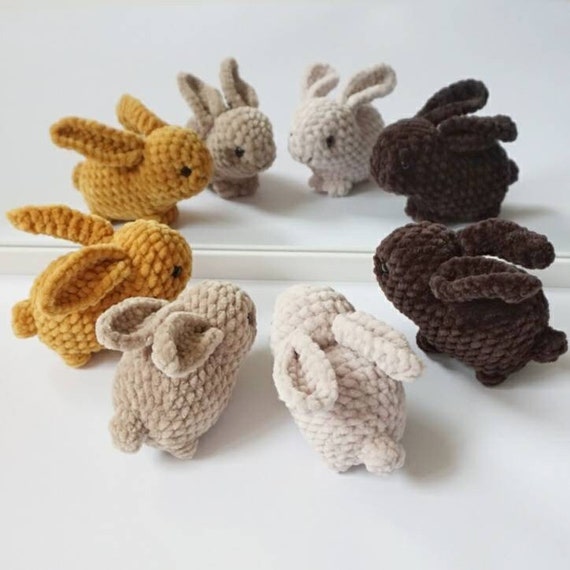The image features a charming assembly of eight small, crocheted bunnies meticulously arranged on a pristine white surface. These adorable bunnies are crafted with fine detail and professionalism, each displaying a consistent circular pattern with a subtle horizontal dividing line running through the center. The bunnies, ovate and fluffy, possess small black eyes and long, gently drooping ears with a noticeable diamond-shaped texture. The color palette includes pairs of dark brown, white, beige, and yellowish hues, each set positioned symmetrically around the circle, giving the impression they are gazing at one another in a quaint, cozy gathering. Their diminutive size suggests they could snugly fit in the palm of one's hand, amplifying their cuteness and the artisanal quality of their creation.